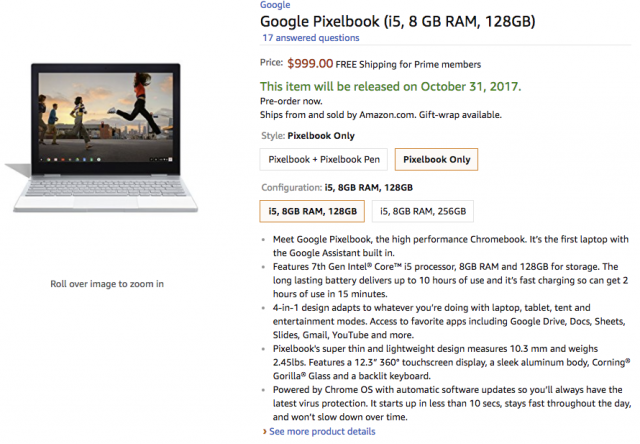The image showcases an Amazon sale page featuring the Google Pixelbook. On the left side of the page, there's a photograph of the laptop, which is turned on. The screen displays an image of four individuals running across a pavement in a cityscape. The person on the far right, likely a woman, is caught mid-air during a leap. She is dressed in a reddish-orange top, jeans, and white sneakers. The backdrop consists of office buildings and taller structures further in the distance, giving an urban feel, though the picture itself is somewhat blurry. The runners are shown in profile from the right side, with the airborne woman leading the group.

On the right side of the sale page, details of the product are displayed:

- **Product**: Google Pixelbook
- **Specs**: Intel Core i5, 8GB RAM, 128GB storage
- **Customer Interaction**: 17 answered questions
- **Price**: $999.00
- **Shipping**: Free for Prime members
- **Availability**: Pre-order now, with the release date on October 31, 2017
- **Seller**: Ships and sold by Amazon.com

The page offers different options for style and configuration:
- **Style**: Pixelbook (highlighted) and Pixelbook Pen.
- **Configuration**: 
  - Highlighted: Intel Core i5, 8GB RAM, 128GB storage
  - Alternate option: Intel Core i5, 8GB RAM, 256GB storage.

Below these selections, additional product details are provided.